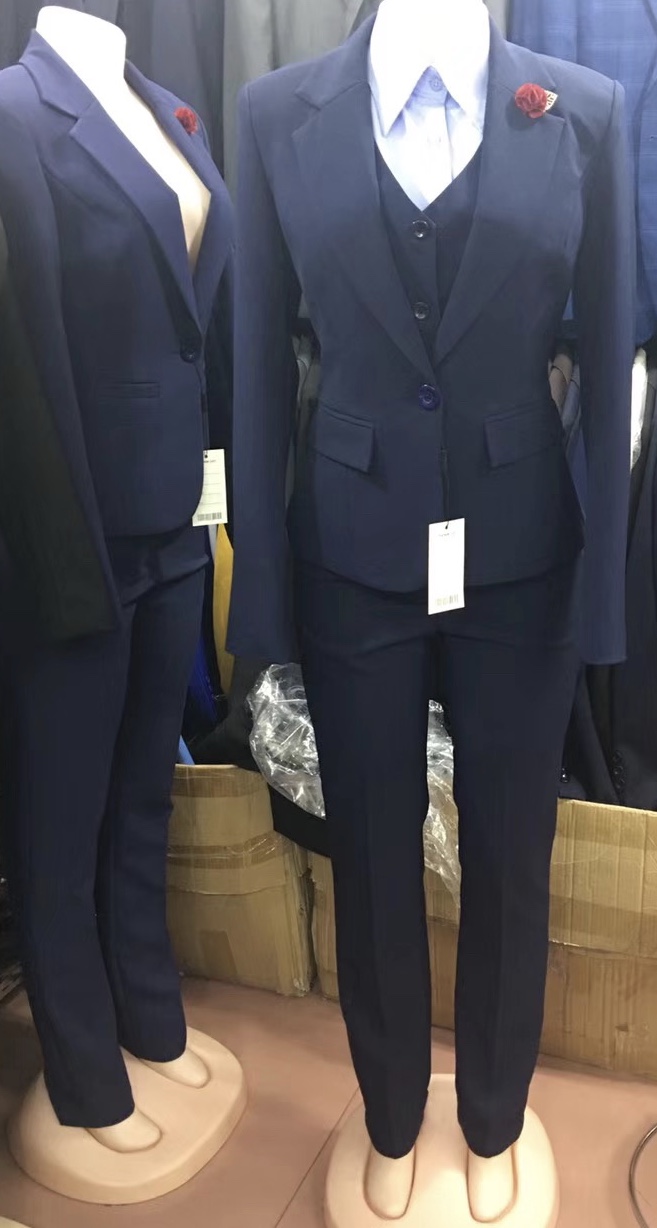The image features two white, headless mannequins dressed in identical, fitted navy blue pantsuits within a women's clothing shop. Each suit consists of a dark navy blue jacket, buttoned at the waist, featuring regular pockets and a matching black vest underneath with multiple buttons, although only two are visible. Beneath the vest, both mannequins are adorned with a crisp, white collared shirt. Elegantly pinned to the left lapel of each jacket is a small red rose or carnation. The mannequins stand on a somewhat cylindrical, pinkish base set against a pink floor. One mannequin faces directly towards the viewer, while the other is turned slightly to the right, adding a dynamic element to the display.